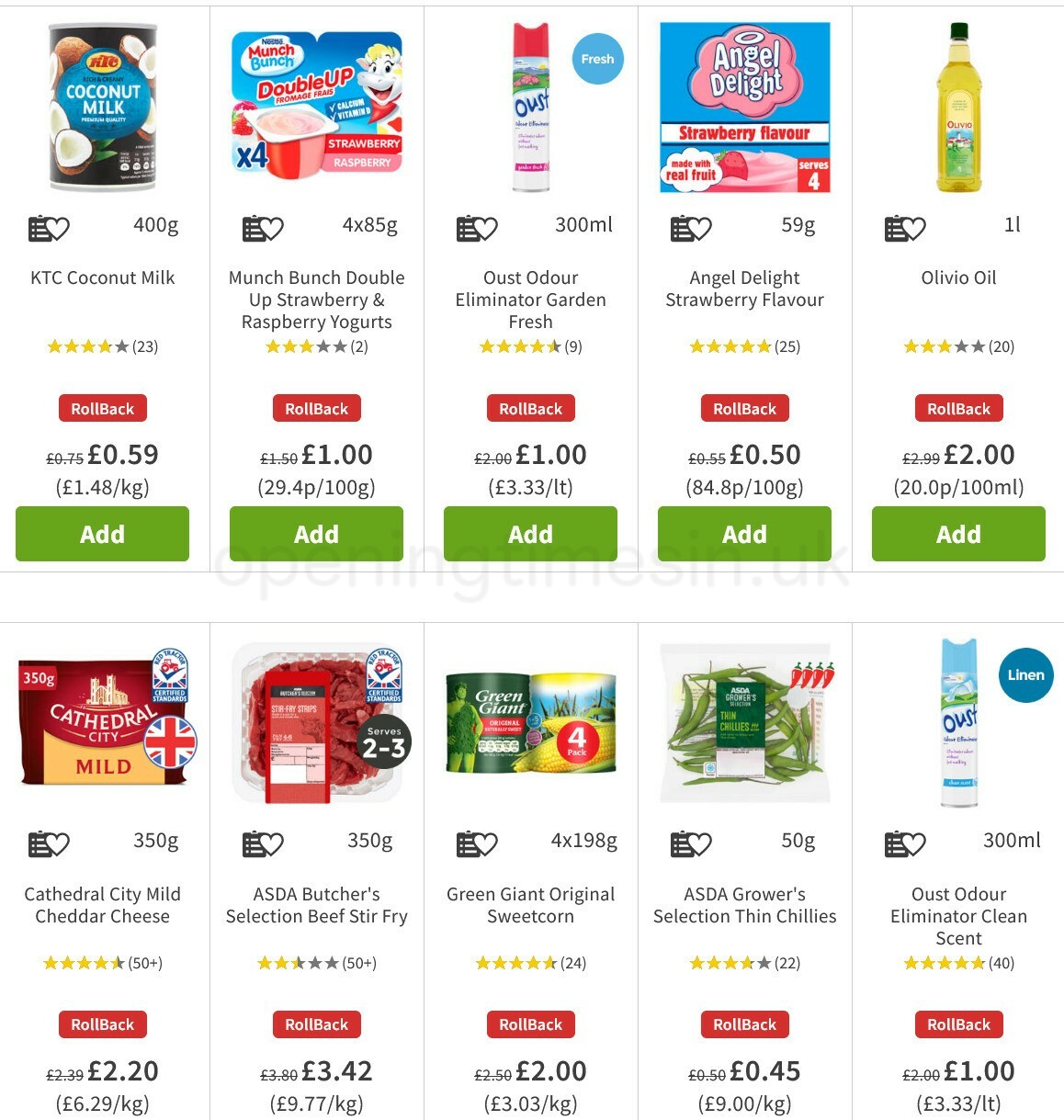The photo showcases a variety of grocery products available for purchase online, displayed against a clean white background. The layout is structured with a thin gray line running horizontally across the top of the image. Five distinct products line up from left to right, each separated by vertical thin gray lines. 

The lower half of the image mirrors this structure, featuring another set of five products, also divided by thin gray lines. Between the two sections, there is an additional thin gray line, a small space, and yet another thin gray line separating the top and bottom rows of products. 

In the center of the image, a faint overlapped stamp reads “opening times and dot UK,” though it is barely visible. Each product is presented with a small photo of the item, accompanied by detailed information. 

For each product, the details are as follows:
- **Top-Left Corner**: A black-bordered calendar icon.
- **Top-Right Corner**: A black-bordered heart icon.
- **Right Side**: Product size (example: “400g”).
  
Below these icons, the product details include:
- **Product Name**: (example: “KTC Coconut Milk”).
- **Rating**: Four yellow stars out of five, with the fifth star in black, followed by "23" in parentheses indicating the number of reviews.
- **Promotional Information**: A red tab with "rollback" written in white.
- **Pricing**: Main price displayed alongside price per kilogram. 
- **Bottom of Product Entry**: A black or green tab with “Add” bolded in white.

Notably, the very last product in the lower row does not include the "Add" tab at the bottom right, distinguishing it slightly from the rest.